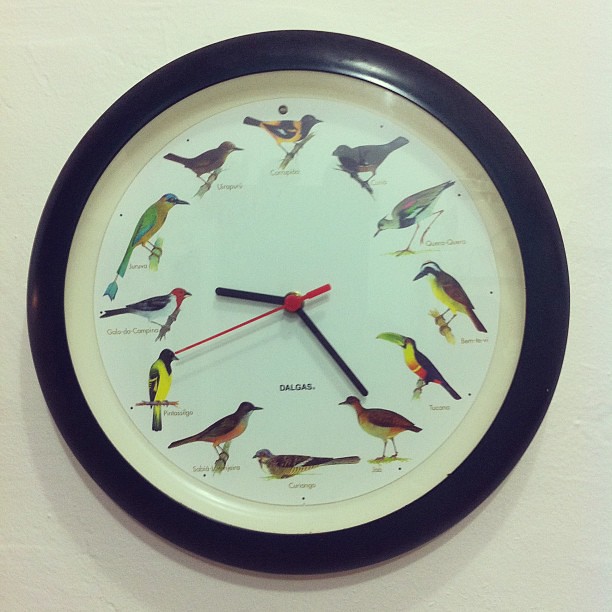Here is a cleaned-up and detailed caption for the image described:

---

This image features an analog clock mounted on a wall. The clock is round with a dark rim, possibly black or dark brown. Enclosed within the rim is a cream-colored circle outlining the face of the clock. Instead of numbers, the clock face has birds positioned where the numbers would typically be, each bird likely representing a particular hour.

At the 12 o'clock position, a bird with a black head, wings, and tail, coupled with an orange chest and breast, is perched on a branch. Moving clockwise, the bird at the 1 o’clock spot is entirely black. The bird at the 2 o’clock position appears to be a type of waterfowl with long legs and a mix of gray, black, white, purple, and green plumage. 

In the 3 o'clock spot, there is a yellow-breasted bird with a brown and black back, a black head striped in white, and a black beak. The 4 o’clock bird is a toucan characterized by a dark back, red and yellow chest, and a long, slightly curved yellow beak. At the 5 o’clock position, a light-breasted bird with a somewhat brownish back and wing features a dark beak and webbed feet, indicating it might be a type of waterfowl.

The 6 o'clock bird is lying down, showing a dark wing with a patterned tip, a white stripe, a grayish head, and a yellowish belly. At 7 o’clock, there's a bird with a dark back, head, and tail, and a reddish to light brown chest. The 8 o’clock bird sports a bright yellow chest, black head and wings with a yellow stripe, and black tail feathers.

Positioned at 9 o’clock is a bird with a dark blue to blackish back and tail with a white tip, a reddish face, and a white chest. The bird at 10 o’clock is tropical, colorful with green and blue plumage, a tail shaped like an arrowhead, a bluish head, yellowish chest, and a gray beak, perched on a stick. Finally, the 11 o’clock bird is brown and is also perched on a stick.

The clock hands show that the time is approximately 9:24. The minute hand points toward the five, the hour hand lies between nine and ten, while the second hand is aligned with the eight. At the bottom center of the clock face, the word "DALGAS" is inscribed, indicating the brand.